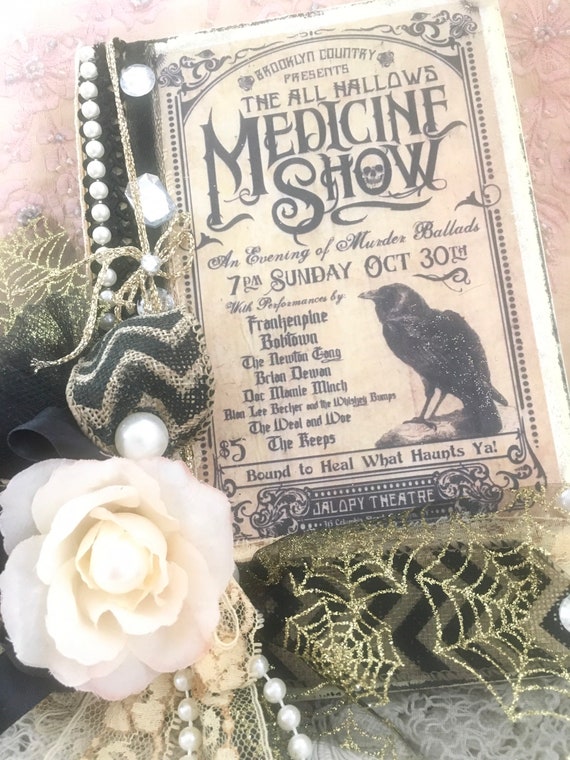The image depicts a detailed and ornate poster for the "All Hallows Medicine Show" presented by Brooklyn County. The show is scheduled for 7 p.m. on Sunday, October 30th, at the Jalopy Theater, promising "an evening of murder ballads" with performances by artists such as Frankenpine, Bobtown, the Newton Gang, Brian Dewan, Dak Marnie Minch, Alan Lee Boettcher, and more. The poster's lively design features an illustration of a black crow perched on a gray log in the bottom right corner. Surrounding the poster, there are various decorative elements: a white artificial flower, a beaded pearl string, and gold spiderwebs set against a light peach or tan background. Additional embellishments include a sparkly spiderweb and a black and gold ribbon on the left side, adding to the overall spooky aesthetic. The font on the poster is spooky, with the "O" in "Show" creatively designed with a skull in its center. The scene exudes a festive, eerie atmosphere perfect for a Halloween-themed event.